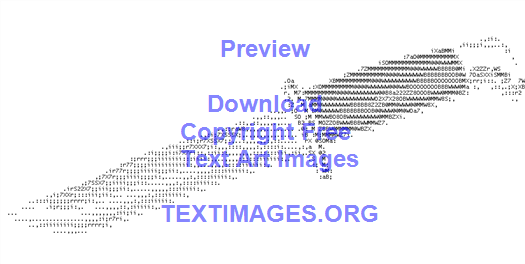This image features a computer-generated sketch of a pocket knife on a white background, created using a series of black and gray letters, numbers, and symbols reminiscent of the output from an old dot-matrix printer. The image includes detailed elements like a black handle and a gray blade, with the design characterized by horizontal lines of black squiggles and white spaces, giving it a textured, pixelated appearance. Superimposed on the knife illustration is bold, light purple text that reads "Preview, Download, Copyright Free, Text Art Images," along with the website "textimages.org" displayed at the bottom. This overlay not only emphasizes the source but also blends into the intricately detailed image of the knife.